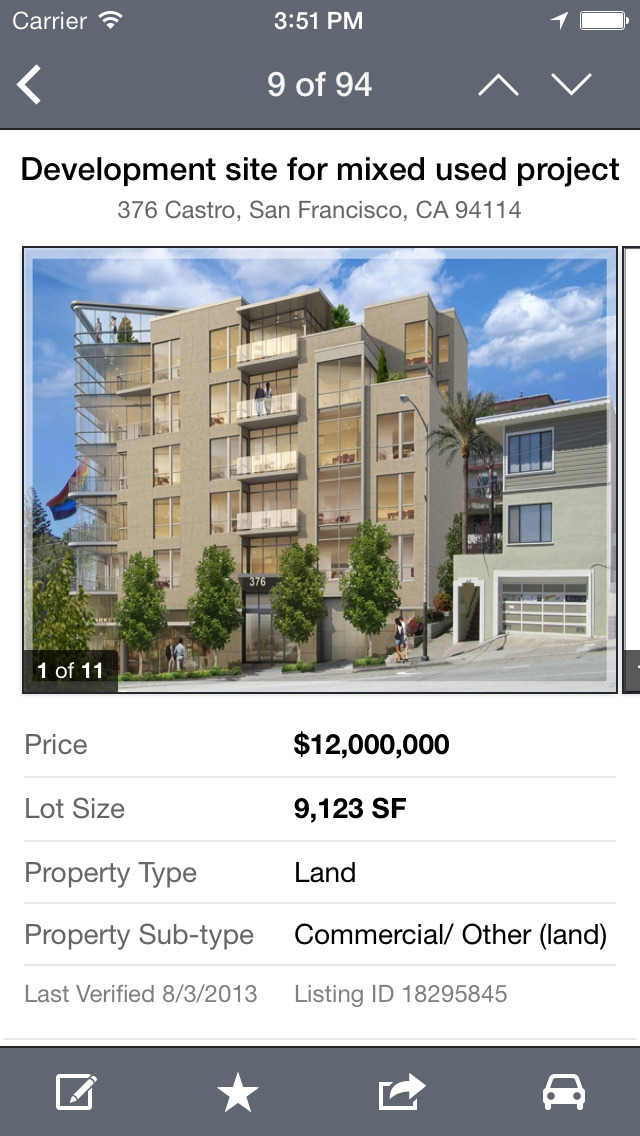A detailed screenshot, taken on a mobile device, showcases the carrier's name, a strong Wi-Fi signal, and a fully charged battery at 100%. The time of capture is noted as 3:51. The location services icon is active, and the screenshot indicates navigation through documents with a status of "9 of 94." Arrows for scrolling up and down are visible.

In the screenshot, details of a development site for a mixed-use project at 376 Castro, San Francisco, California, 94114 are prominently displayed. The image features an artistic rendering of a modern six-story residential building. The exterior is depicted with sleek, contemporary design elements. Surrounding the building are lush palm trees and additional greenery, enhancing the area's aesthetic.

It’s one of 11 photos provided in the listing, which suggests a scenic and comprehensive portrayal of the property. The asking price is listed at $12 million, and the lot size is documented as 9,123 square feet. The property is classified as land, indicating it is likely still under development or being sold primarily for its future potential.